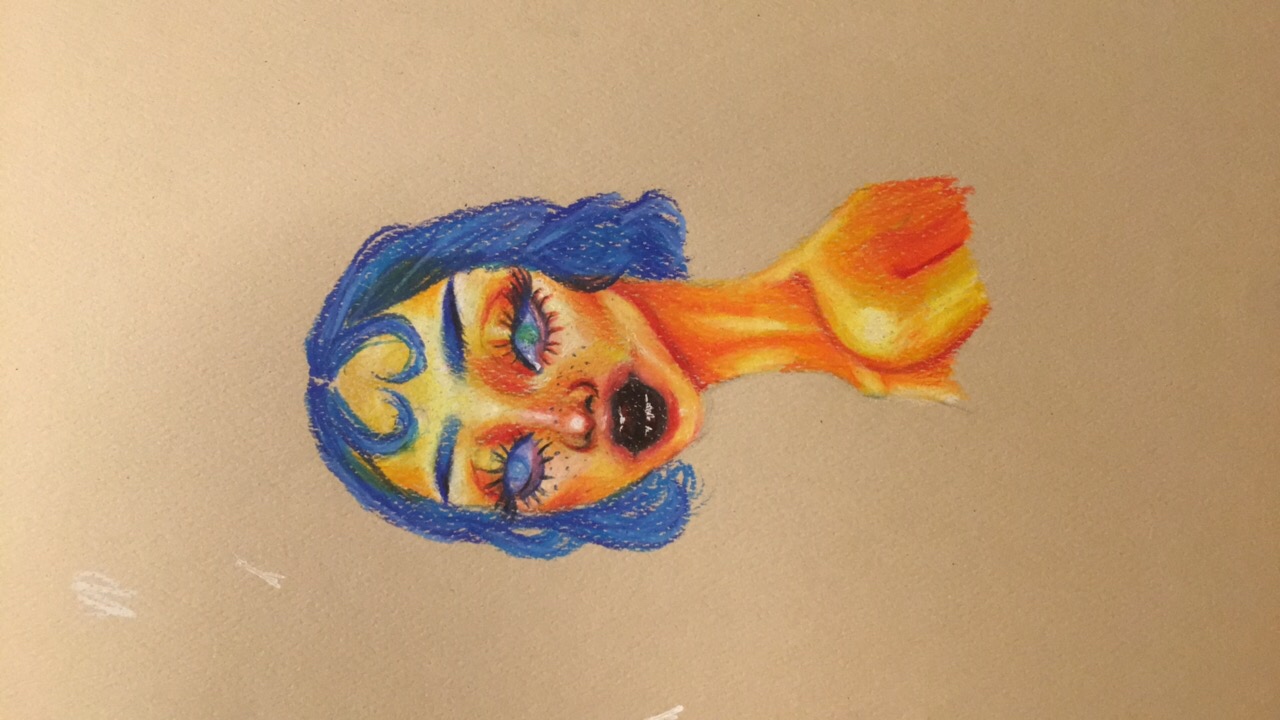The image features a detailed drawing, likely done with pastel pencils, of a woman depicted from her shoulders up. This woman has a slender build, with a long neck and prominent collarbone visible on her left-hand side. Her upper body is turned slightly to the left, with the shoulders tilted forward. The right side of her shoulder and a portion of her upper arm is clearly visible. She gazes directly at the viewer with large, light blue eyes adorned with big, mascara-coated eyelashes. Her facial features are meticulously detailed, with a well-drawn nose and freckles speckled across her tan or yellowish-orange skin. The woman’s mouth is open, revealing white teeth, and her lips are painted a dark, almost black color.

Her hair is entirely blue, kept short and slightly wavy, ending just around her chin. The hair is parted in the middle, and two elegant curls frame her forehead, forming an upside-down heart shape. Her blue eyebrows transition to black at the ends, adding a striking contrast to her facial expression. The image is set against a brown, textured background that is lighter at the top and darker at the bottom, with a couple of white chalk or pastel scribbles in the upper left corner giving it an artistic touch.